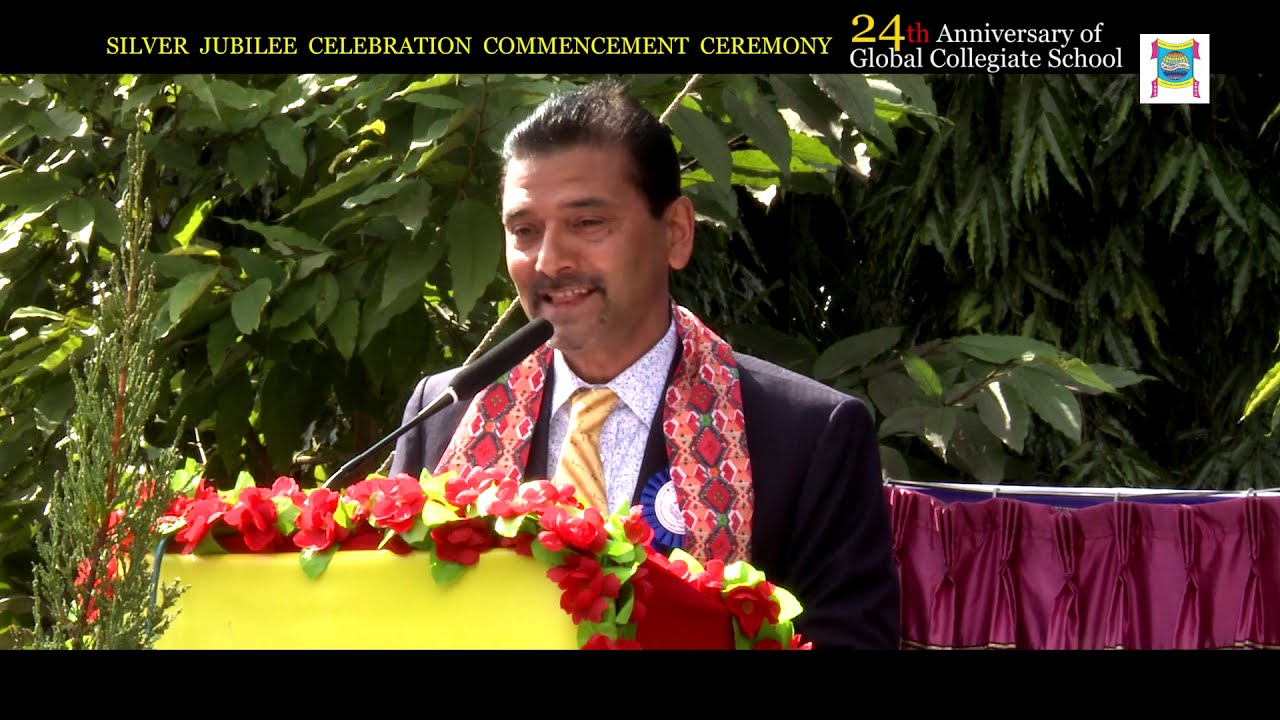In this vibrant scene captured outdoors, a man with short black hair and a thin mustache stands at the center, passionately addressing the audience from behind a yellow podium adorned with an arrangement of pink and red flowers and yellow-green leaves. Dressed in a gray suit, a patterned white shirt, and a yellow and red striped tie, he engages the crowd through a narrow microphone. The backdrop features a purple curtain, partitioning another area and accentuated by large green palm leaves and other lush foliage, suggesting an outdoor setting. Thick horizontal black borders frame the image, with the top border displaying in bold, yellow capital letters, "Silver Jubilee Celebration Commencement Ceremony," and just below in white letters with the number "24" in yellow, "24th Anniversary of Global Collegiate School." The image captures the moment, likely a commencement speech, celebrating a significant milestone for the institution amidst a sunny, tree-filled background.